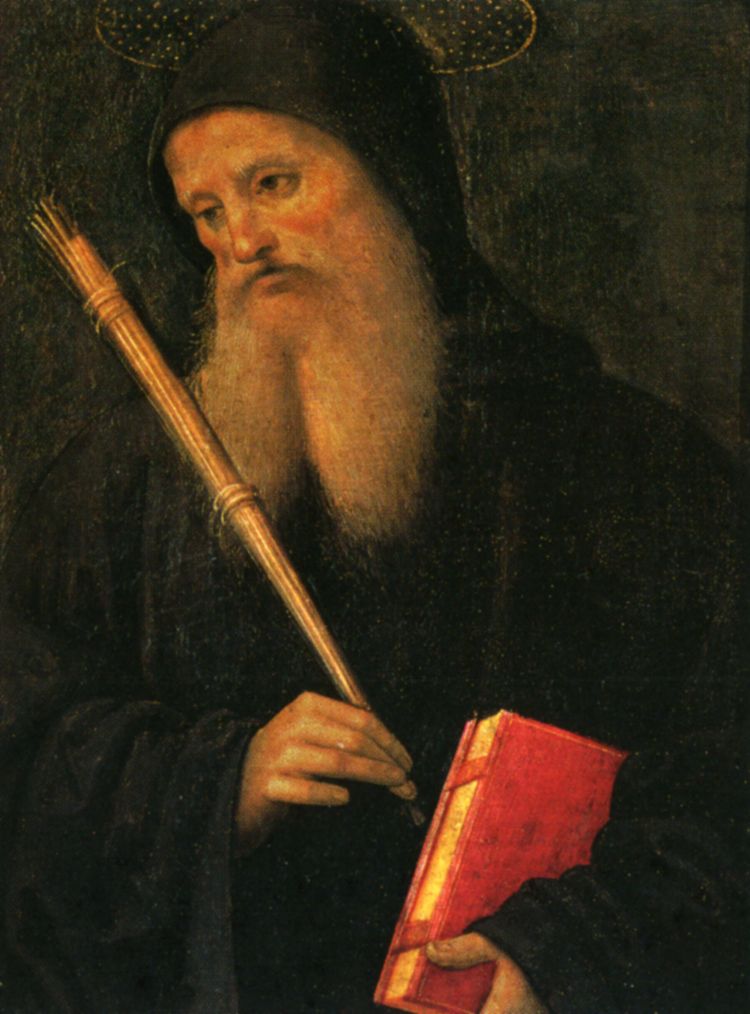The detailed painting captures an older Caucasian man with a somber expression, his head tilted slightly to the left. He is dressed in a long black robe that envelops his entire body, except for his hands and face. His most distinguishing feature is a long white beard, parted in the middle into two sections, and a black hood drapes over his head. The man's dark brown eyes suggest a contemplative mood.

In his left hand, he grasps a golden tube-like device, angled towards the top left corner of the painting, while his right hand cradles a red, leather-bound book adorned with red straps and clasps, revealing yellowed pages. This book suggests both age and significance, possibly holding religious or scholarly texts. The backdrop is a dark gray, creating a somber and introspective atmosphere for the figure.

Subtle golden circular shapes with dotted centers appear near the figure's head, reminiscent of a halo or other religious symbolism, which enhances the mystical quality of the artwork. Painted in watercolor on canvas, this evocative portrait, though unsigned, likely represents a religious or scholarly figure and evokes a sense of reverence and introspection.